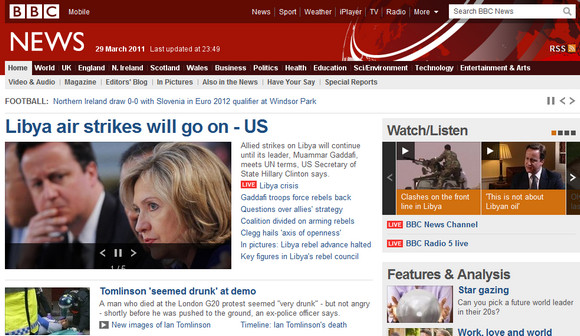Screenshot of the BBC News Mobile page from 29th March 2011, last updated at 23:49. At the top, a dark maroon banner displays the BBC Mobile logo alongside menu options for News, Sport, Weather, iPlayer, TV, Radio, or more, and a search bar stating 'Search BBC News'. Below, a red banner reads, "NEWS, 29 March 2011, last updated at 23:49," and includes the BBC World News icon and an orange RSS icon.

A black navigation bar below features sections such as Home (which is selected), World, UK, England, Northern Ireland, Scotland, Wales, Business, Politics, Health, Education, Science & Environment, Technology, and Entertainment & Arts. Under the Home selection, a light blue sub-menu includes options like Video & Audio, Magazine, Editor's Blog, In Pictures, Also in the News, Have Your Say, and Special Reports.

The main content of the page begins with a football update: "Northern Ireland draws 0-0 with Slovenia in Euro 2012 qualifier at Windsor Park." Below, a prominent headline states, "Libya airstrikes will go on - US," accompanied by an image of two American politicians. The news details that allied strikes on Libya will continue until its leader, Muammar Gaddafi, complies with UN terms, according to US Secretary of State Hillary Clinton. A red 'LIVE' button and a 'Libya Crisis' selectable field are nearby.

Additional linked headlines under the Libya news include:
- Gaddafi troops force rebels back
- Questions over allies' strategy
- Coalition divided on arming rebels
- Clegg hails 'axis of openness'
- In pictures: Libya rebel advance halted
- Key figures in Libya's rebel council

Another article titled "Tomlinson seemed drunk at demo" follows. An unclear image shows yellow, blue, and white hues with a person seemingly either lying down on the ground or a bench. The caption mentions that the man who died during the London G20 protest appeared very drunk rather than angry shortly before being pushed to the ground, according to an ex-police officer. Selectable fields for "New images of Ian Tomlinson" and "Timeline: Ian Tomlinson's death" are offered below.

On the right side, under 'Watch/Listen', two videos are available: "Clashes on the front line in Libya" and "This is not about Libyan oil." Further options include live streams for the 'BBC News Channel' and 'BBC Radio 5 live.' Features and analysis sections highlight articles such as "Stargazing: Can you pick a future world leader in their 20s?" and another partially visible title, "Work, love, and world."